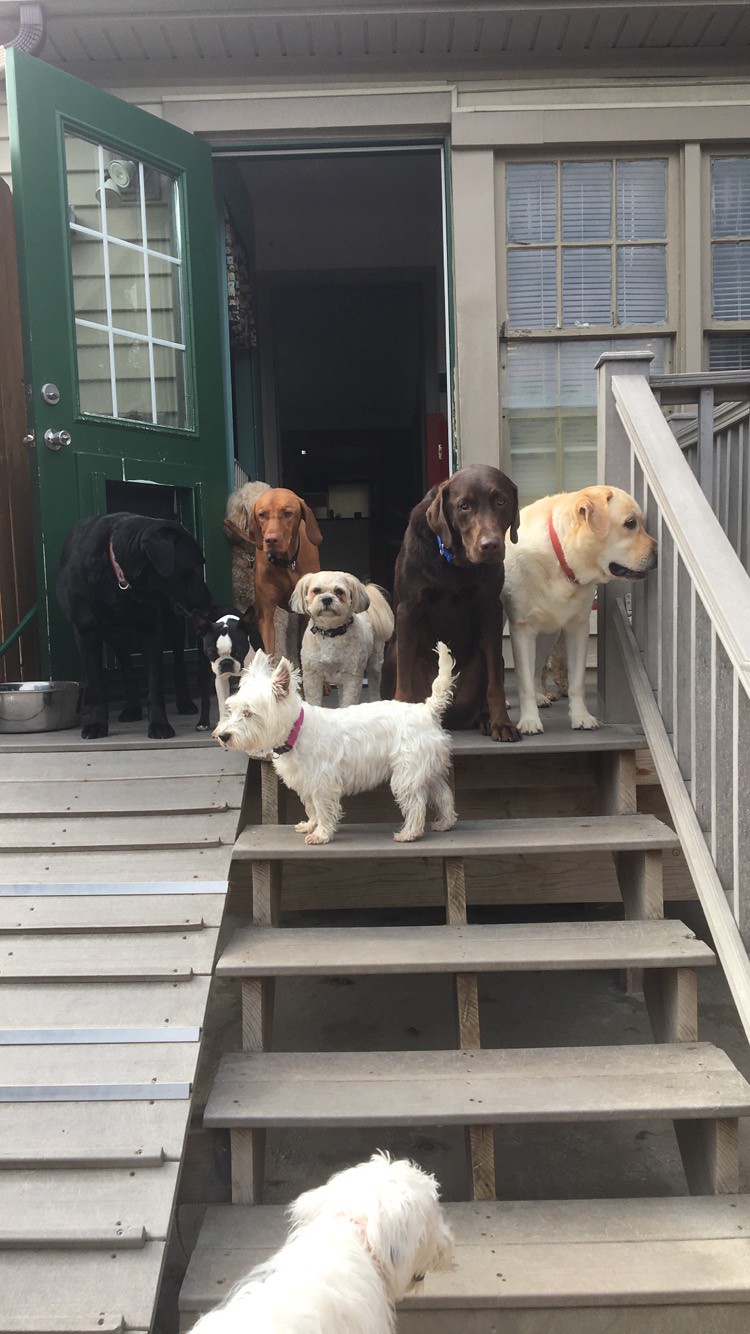A diverse group of nine dogs of various sizes and breeds, including poodles, westies, hound dogs, a yellow lab, a chocolate brown dog, and black dogs, stand on a wooden porch with stairs leading down and a ramp to the side. The dogs' colors range from black, chocolate brown, yellow, to white. Most of the dogs are gathered at the top of the stairs, while a small white dog, likely a westie with a pink collar, is on a lower step, appearing to be climbing up. Another white dog is partially visible at the bottom of the steps. One black dog with a collar stands at the foot of the ramp. There's also a metal dog bowl near the ramp. The backdrop features a light-colored house with a green door that has a steel doorknob and a window at the top. The door is open, allowing the dogs to freely move in and out, and there is a partial view of a dog door. The scene suggests a welcoming, pet-friendly environment with plenty of space for the dogs to socialize and play.